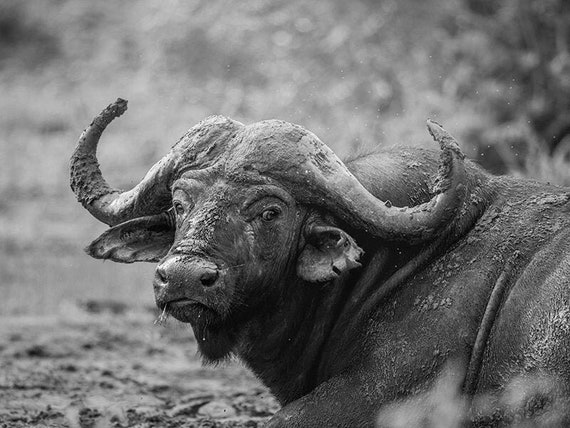In this striking black-and-white photograph, a water buffalo reclines serenely in a muddy terrain, gazing back over his shoulder at the viewer with large, slanted eyes. His rough hide is extensively caked in mud, particularly on his back, neck hump, and large, upward-curving horns. A bit of straw dangles from his mouth, suggesting a relaxed state, further emphasized by his downturned, relaxed ears. His snout and the flap of skin under his chin also bear traces of mud. The ground around him is thick with mud, its texture accentuated by the image's high contrast. The background, in stark contrast, is soft and flooded with light, rendering it hazy and unclear, with only a hint of vegetation. Despite his bedraggled appearance, the buffalo exudes a sense of calm and unbothered tranquility, comfortably ensconced in his muddy surroundings.